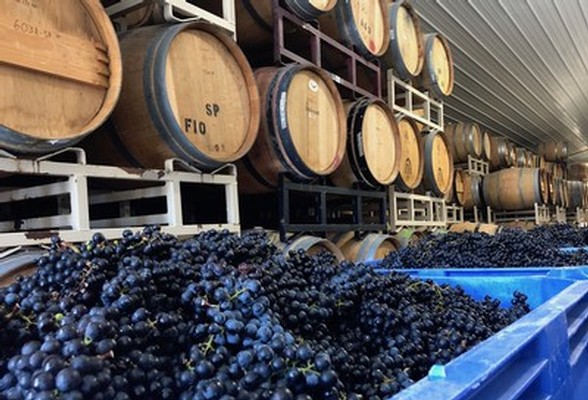This detailed image depicts an indoor winery or wine distillery bathed in natural light. The setting features large blue plastic containers overflowing with ripe purple and black grapes, ready for wine production. Wooden barrels, meticulously arranged on white platforms, line the left side of the space. There are ten barrels facing outward, organized in a two-row configuration—six on the first row and four on the second, stacked above. Additionally, several barrels are positioned on top of crates, one of which is labeled 'F10SP.' The white roof of the building, with prominent horizontal ribs, is clearly visible and adds to the industrial ambiance. Overall, this well-organized space is dedicated to the intricate process of winemaking.